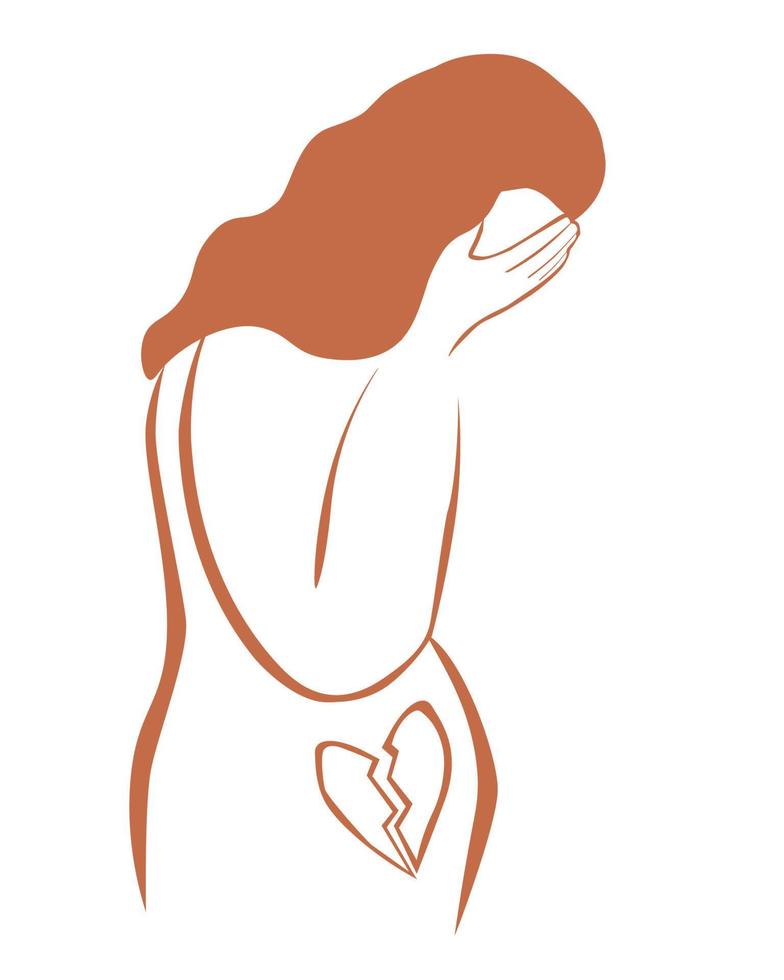The image is a minimalist cartoon drawing of a distressed woman, characterized by its use of a singular dark pink-orange color. The drawing presents a silhouette-like outline of the upper half of the woman's body, extending slightly past her hips. Her head is bowed down in sorrow or shame, obscured by her long, solid-colored hair, and she is holding her face in her hands, conveying profound sadness. Notably, her posture suggests she might be crying. Her skin is depicted as starkly white, enhancing the emotional impact of her sorrowful demeanor. A prominent feature of this image is the visual representation of a broken heart in her swollen belly, hinting at a likely pregnancy loss or impending emotional trauma. The broken heart, illustrated as two halves separated by a jagged line, is drawn with the same dark pink-orange color, symbolizing deep anguish. There are no words in the image, leaving the viewer to infer the woman's profound grief and heartbroken state through her body language and the simple, yet powerful symbols.